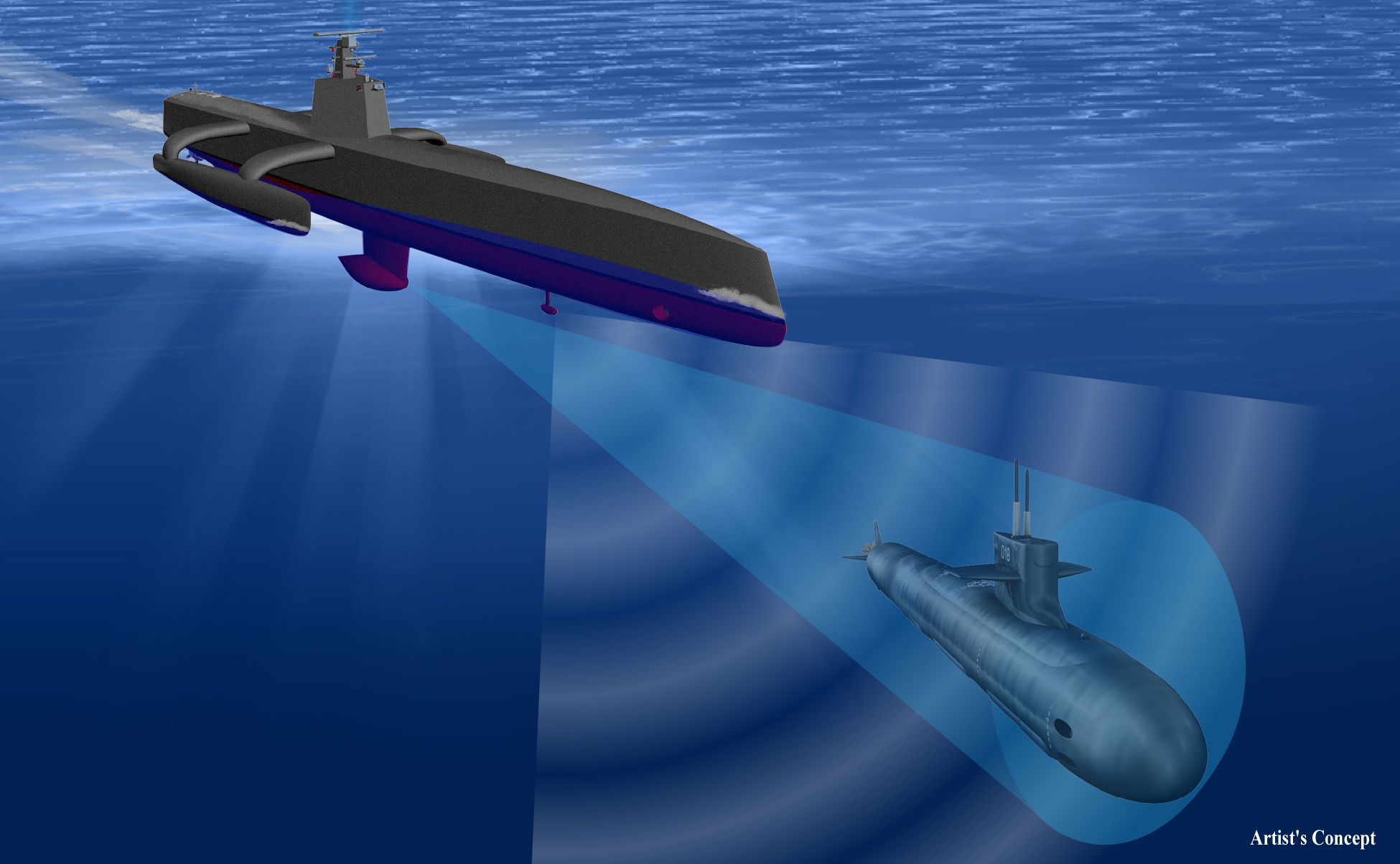This detailed digital artwork portrays a 3D-rendered scene beneath the ocean’s surface, featuring two submarines. The top submarine, colored in gray and purple, is larger and equipped with sophisticated tracking technology, potentially using sonar or infrared scanning, as indicated by the beams of light spreading throughout the water. This submarine seems to be engaged in a search or rescue operation, possibly locating the smaller, light blue submarine positioned below it on the right. Both submarines exhibit distinct designs and shapes, contributing to the dynamic underwater tableau set against the backdrop of the deep blue ocean. The artwork captures the tension and precision of underwater navigation and surveillance, marked as an artist’s conceptualization in the corner, suggesting a creative interpretation rather than a literal depiction.